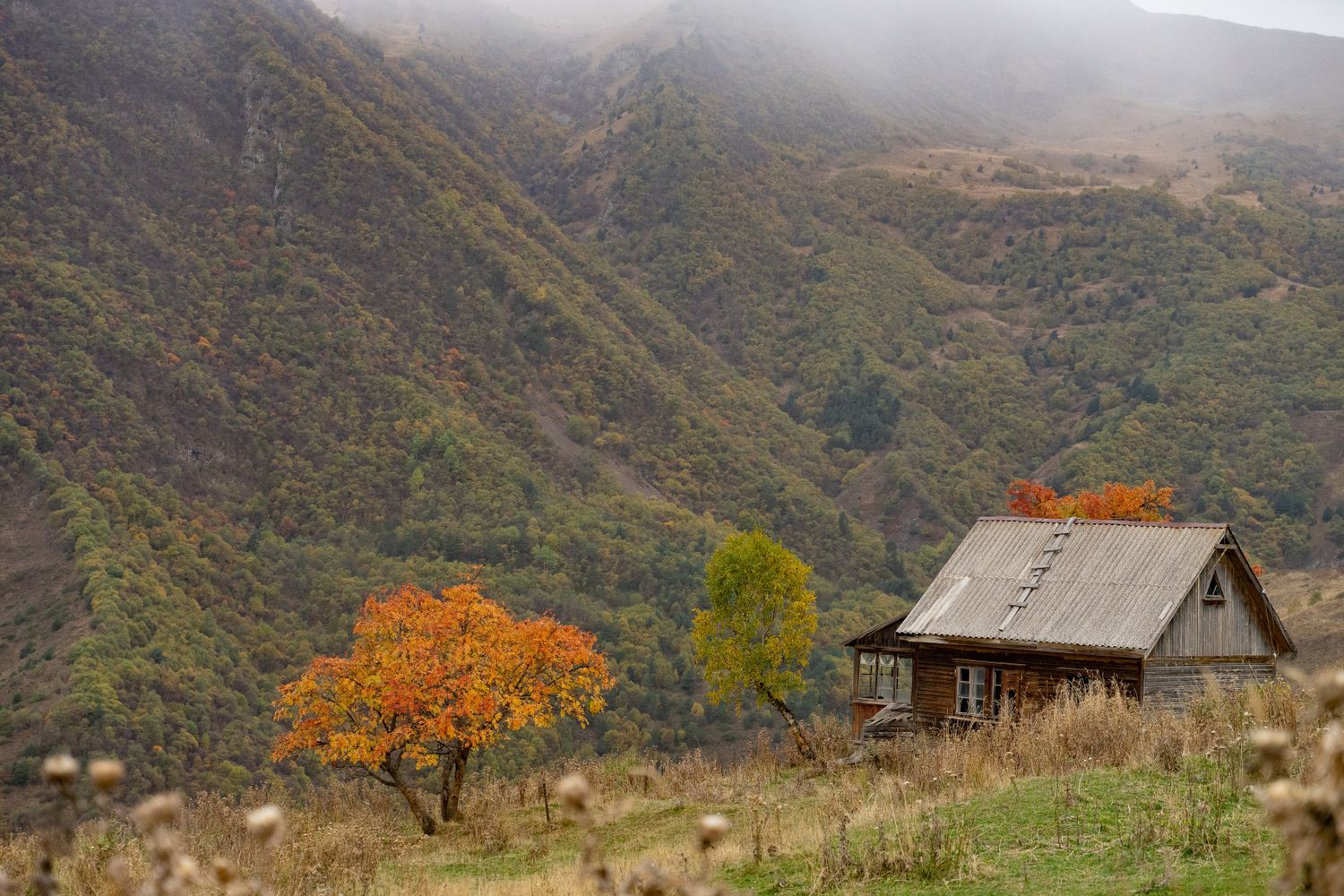This is a detailed landscape photograph captured from an elevated vantage point, depicting a serene mountain cabin scene. The viewer looks across a lush valley towards relatively tall, wooded mountains whose mist-covered tops create a mystical ambiance. The mountains feature a series of ridges and pathways, giving a sense of depth and grandeur. 

In the foreground, a picturesque wooden cabin with a metal roof, distinctive for its glassed-in front porch and a peculiar ladder-like structure on the roof, offers a charming focal point. The cabin, made of logs, includes several windows, one of which is triangular, adding to its rustic appeal. The structure sits amidst an array of tall, overgrown grasses and wildflowers, accentuating the untamed beauty of the landscape.

Surrounding the cabin, the trees display a vivid palette of fall colors. A prominent green tree is beginning to turn yellow, while another in the foreground has fully transitioned to bright orange. Additionally, there is a larger tree with an orange canopy and a brown trunk, emphasizing the autumnal theme. The overall scene, viewed from a perspective slightly above the cabin’s roof, suggests that the cabin offers stunning views of the scenic, mountainous backdrop.